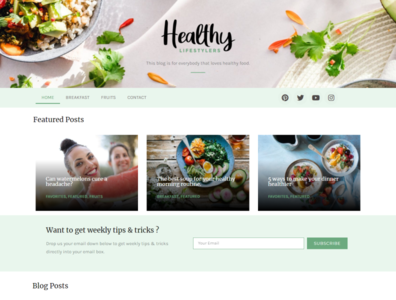In the image, we observe a webpage belonging to a site called "Healthy." The image quality is extremely blurry, making it challenging to discern the finer details. At the very top of the page, the word "Healthy" is prominently displayed in cursive black text. Directly beneath it is the word "Lifestyles" in green text.

Below the "Healthy Lifestyles" header, there is additional text that remains illegible due to the blur. The navigation menu includes options such as "Home," "Breakfast," an indiscernible item, "Contact," and an array of social media icons on the right, including Facebook, Twitter, YouTube, and Instagram.

Beneath the main navigation, there is a section titled "Featured Posts" in black text. This section showcases three images, each accompanied by white text with green subtext, although specific details of the text are obscured by the blurriness.

Further down, there is a call-to-action section that reads "Want to get weekly tips and tricks?" accompanied by a text field labeled "Your email" and a green button that says "Subscribe." Below this segment, the page lists "Blog Posts."

The background of the "Healthy" logo features a bowl containing a mix of rice, various greens, and perhaps carrots, positioned on a white table slightly left of center. The first image in the "Featured Posts" section depicts two women smiling while eating watermelon. The second image showcases a colorful salad with avocado, eggs, broccoli, tomatoes, and an assortment of other vegetables. The final image presents two bowls of what appears to be a white cream, possibly ice cream, garnished with vegetables or similar toppings.